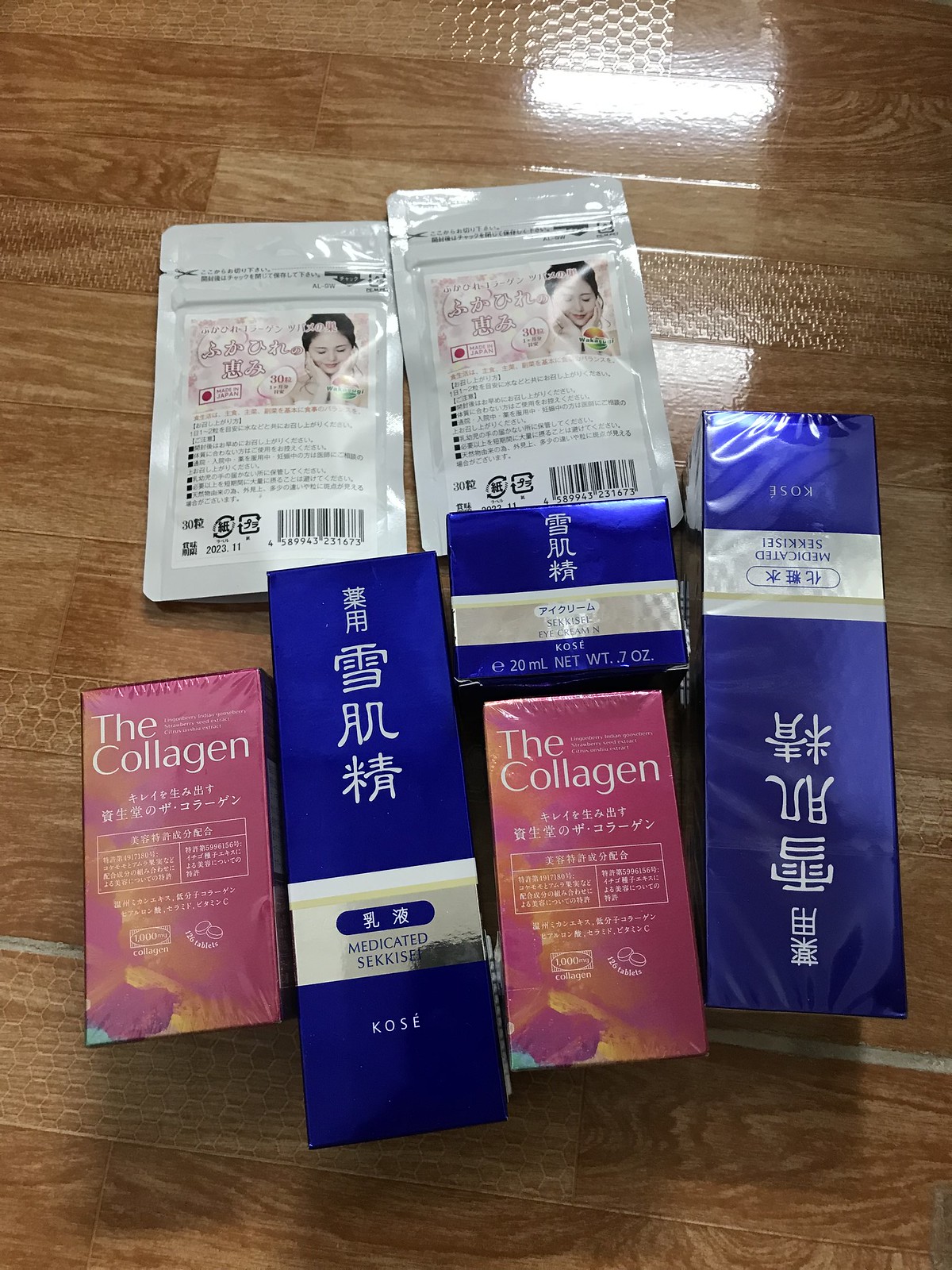In this image, a selection of five boxed Korean beauty care products is artfully arranged on what appears to be a medium brown, wood-grain surface, possibly a wooden table or hardwood floor featuring some geometric patterns. The assortment includes two reddish-orange boxes labeled "The Collagen" in white font, with accompanying Korean script that is unreadable. Alongside these, there are three metallic bright blue boxes. The leftmost blue box displays large characters and appears to read "medicated something cosay" in English beneath the Korean. The central blue box shares a similar design but is smaller and square-shaped. The rightmost blue box mimics the one on the left but is positioned upside down and wrapped in a protective film, unlike its twin. Positioned above these boxes, two packets, likely containing face masks, feature black and white Korean text with hints of pink in the logo and have resealable tops. The overall arrangement and varied packaging create a visually engaging display of Korean skincare products.